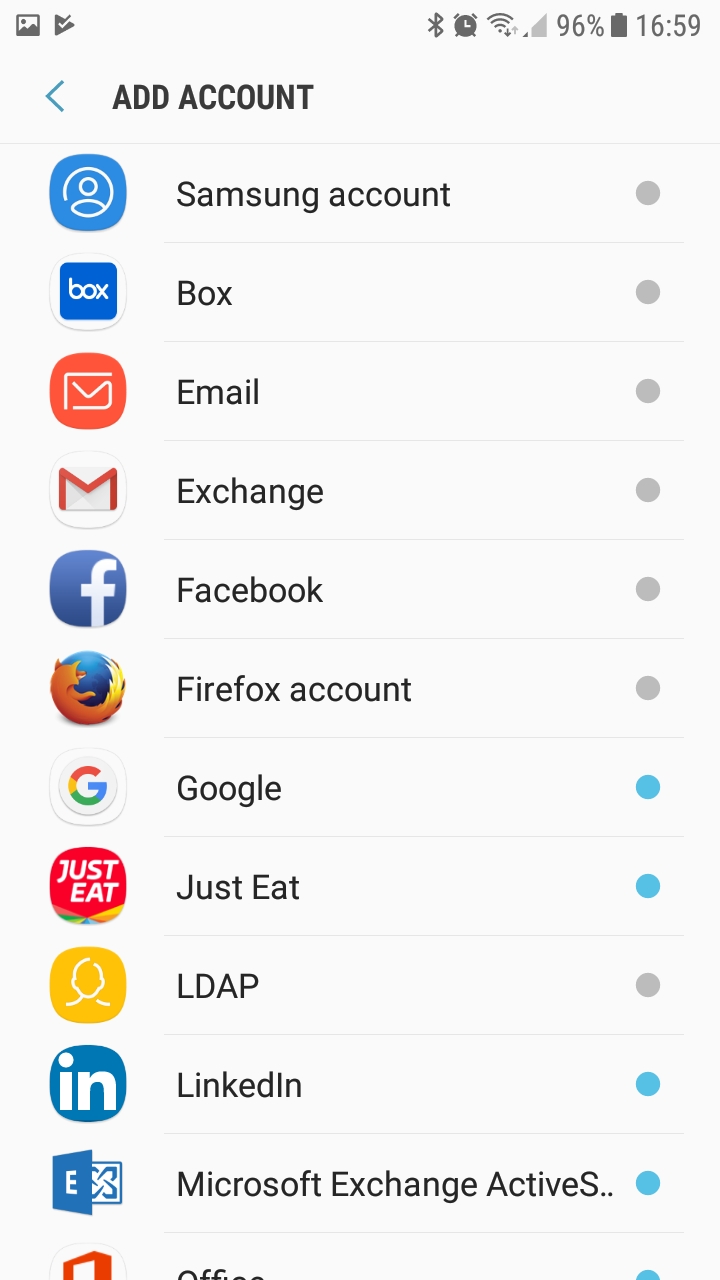A digital screenshot features a pristine white background. The top-right corner displays a battery icon at 96% and a timestamp of 16:59. Adjacent icons include an alarm clock and a Bluetooth symbol. Below these, a comprehensive list of accounts is visible, each marked by a circular checkbox. The list includes:

- Box: grey
- Email: grey
- Exchange: grey
- Facebook: grey
- Firefox Account: grey
- Google: blue
- Just Eat: blue
- LDAP (in all caps): grey
- LinkedIn: blue
- Microsoft Exchange Active (with 'S' and 'A' capitalized): grey
- Office: blue

Each checkbox denotes the status of the account, with grey indicating inactive or unchecked, and blue suggesting active or selected.